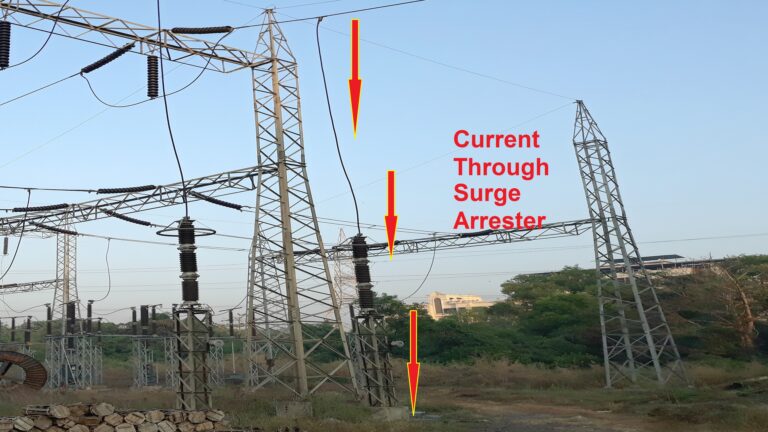The image depicts a power station situated in a clearing amidst a forested area with grass and small trees surrounding it. Central to the scene are multiple metal scaffolding structures supporting power lines that stretch to either side of the image, connecting to other towers in the background. Prominent within the image are three red arrows pointing downward towards a section labeled "current through surge arrester" in red text. This labeling and alteration appear to illustrate the flow of current through a grounding mechanism at the base of the metal structures. The station consists of numerous electrical devices, some silver and black, which are grounded, and connected by cables and wires. Additionally, a chain-link fence encloses part of the area, and a dirt access road runs nearby. The setting is illuminated by daylight, under a clear blue sky, with trees and two buildings visible in the distant background.